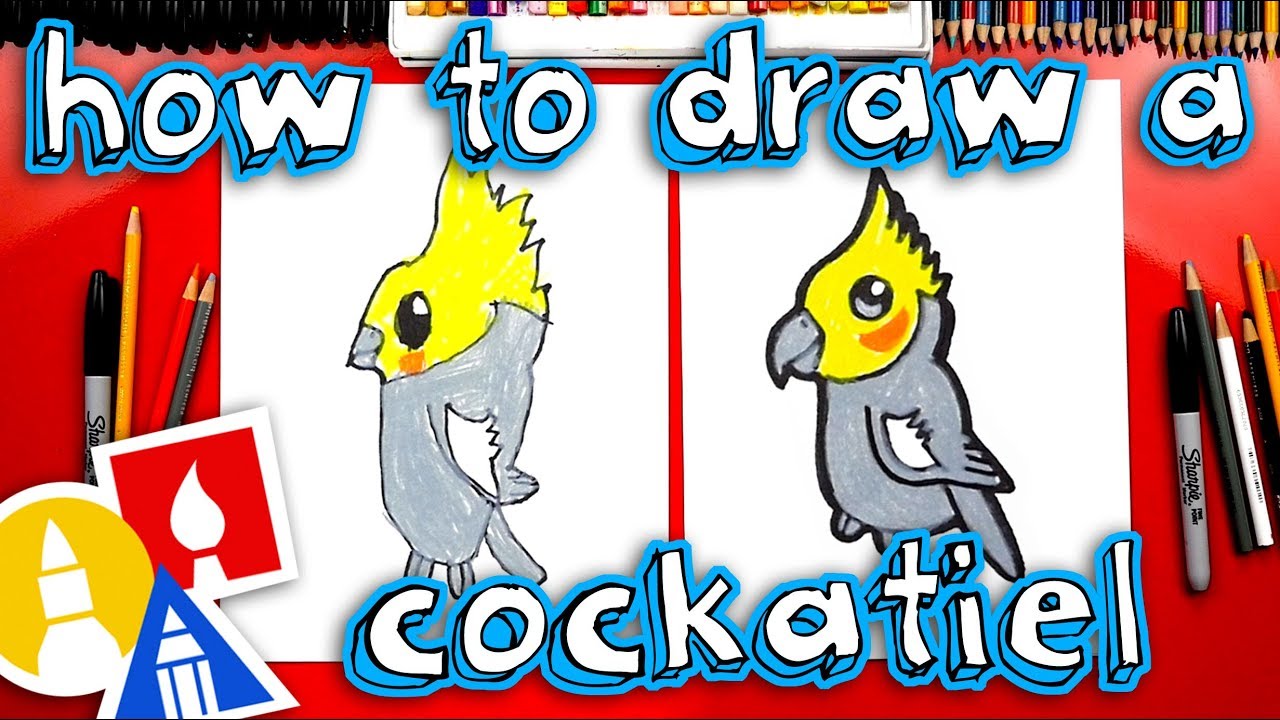The rectangular poster, nearly twice as long as it is tall, features a predominantly red background. Across the top border, art supplies are neatly arranged, with black marker caps on the left, a box of colorful markers in the middle, and the tips of colored pencils lining the right. The right side of the image also shows a Sharpie and various colored pencils, mirrored by similar supplies on the left side. 

In bold, fancy block letters with a white front and blue shadow, the top of the poster reads "how to draw a," while at the bottom, it says "cockatiel." Positioned centrally are two white pieces of paper standing vertically. Each paper showcases a drawing of a cockatiel. The left drawing appears amateurish, with disproportionate features such as a misshapen head and a straight, unslanted back, giving it an unfinished look. In contrast, the right drawing appears more professional, with a realistic eye and beak, and properly curved wings. The cockatiel in both illustrations features a gray body, yellow head, and an orange patch below its eye.

In the bottom-right corner, there's a logo composed of a blue triangle, red square, and yellow circle, each containing white cutout drawings of the top of a colored pencil, a marker, and a paintbrush. Overall, the poster effectively compares an amateur drawing of a cockatiel with a more polished, professional version, accentuated by the various art supplies used to create these renditions.